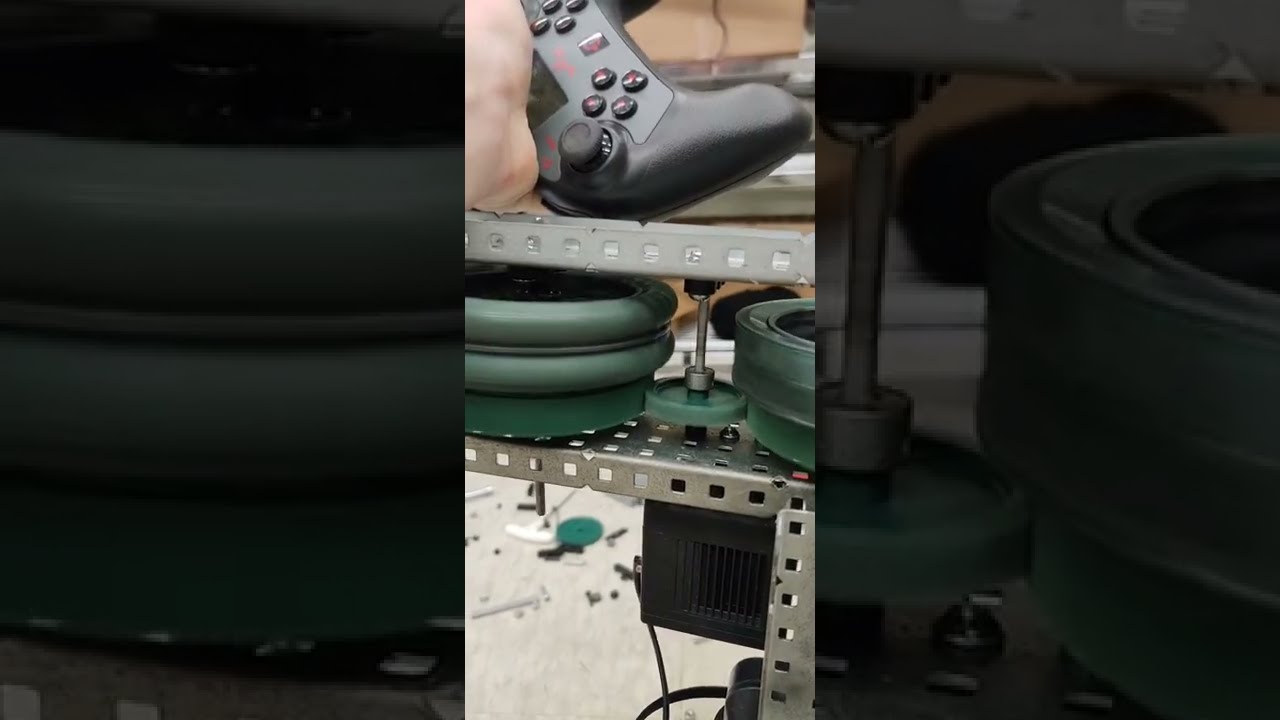This image appears to be a close-up shot within a workshop, featuring a Caucasian hand holding a gray video game controller, possibly for a PlayStation. The hand and controller are positioned atop an industrial work table composed of gray metal, resembling an erector set style shelving unit. Two shelves are held together by a jack mechanism, which has three green disc rings on either side for support. Scattered tools and scraps can be seen on the floor beneath the table, along with an electrical transformer bolted to the lower portion of the apparatus. The image is an incomplete or partial shot, with the left and right borders darkened and enlarged portions of the original photo, emphasizing the green circles. The overall setting likely reflects a workspace where equipment is either being built or repaired.